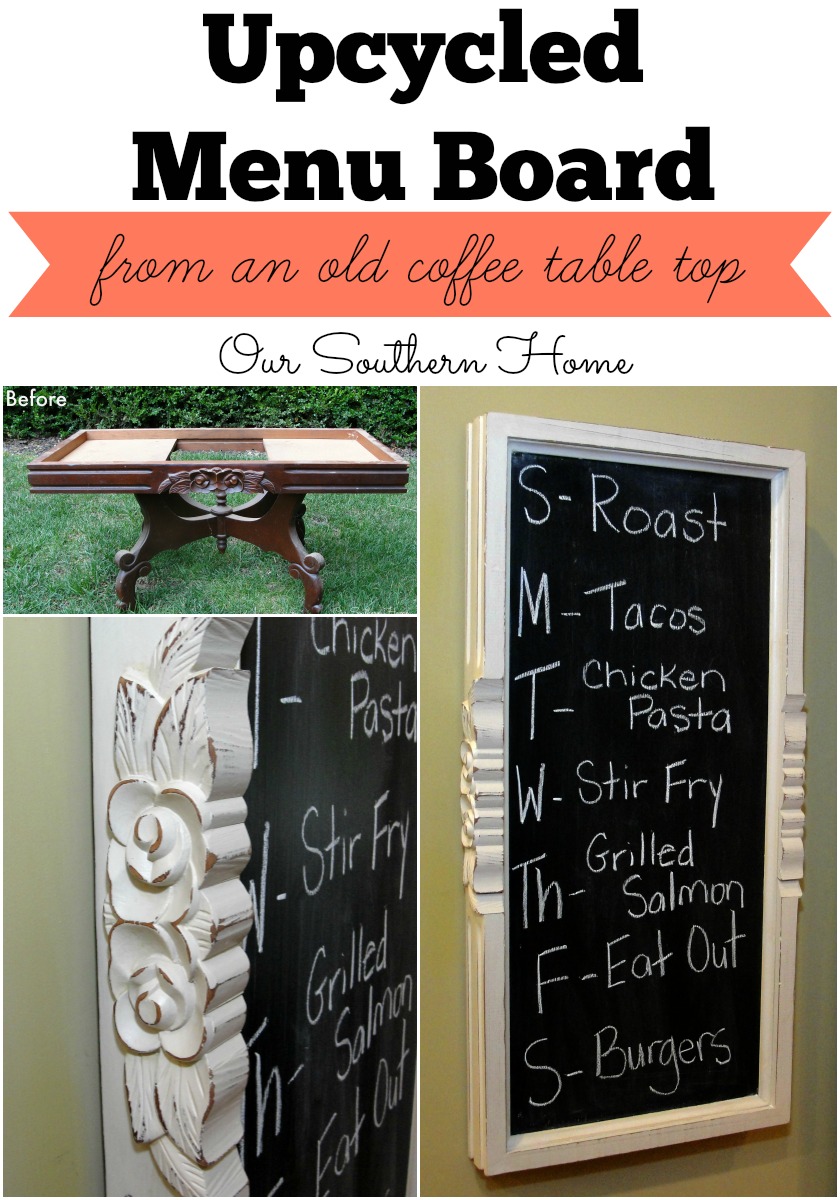The image is titled "Upcycled Menu Board" in bold black text against a white background. Below, an orange ribbon with black script reads, "from an old coffee tabletop," followed by "Our Southern Home" in black text on a white background. The collage consists of three photographs: the top left shows a 'before' image of a brown, ornately carved wooden coffee table sitting on a grassy lawn. The two lower photos show the 'after' transformation, where the table has been upcycled into a menu board. The repurposed board, now painted white around the edges, hangs on a wall with a blackboard center. Written in chalk are daily menu items: S (Sunday) Roast, M (Monday) Tacos, T (Tuesday) Chicken Pasta, W (Wednesday) Stir Fry, TH (Thursday) Grilled Salmon, F (Friday) Eat Out, S (Saturday) Burgers. The days of the week are neatly listed down the left side of the board.